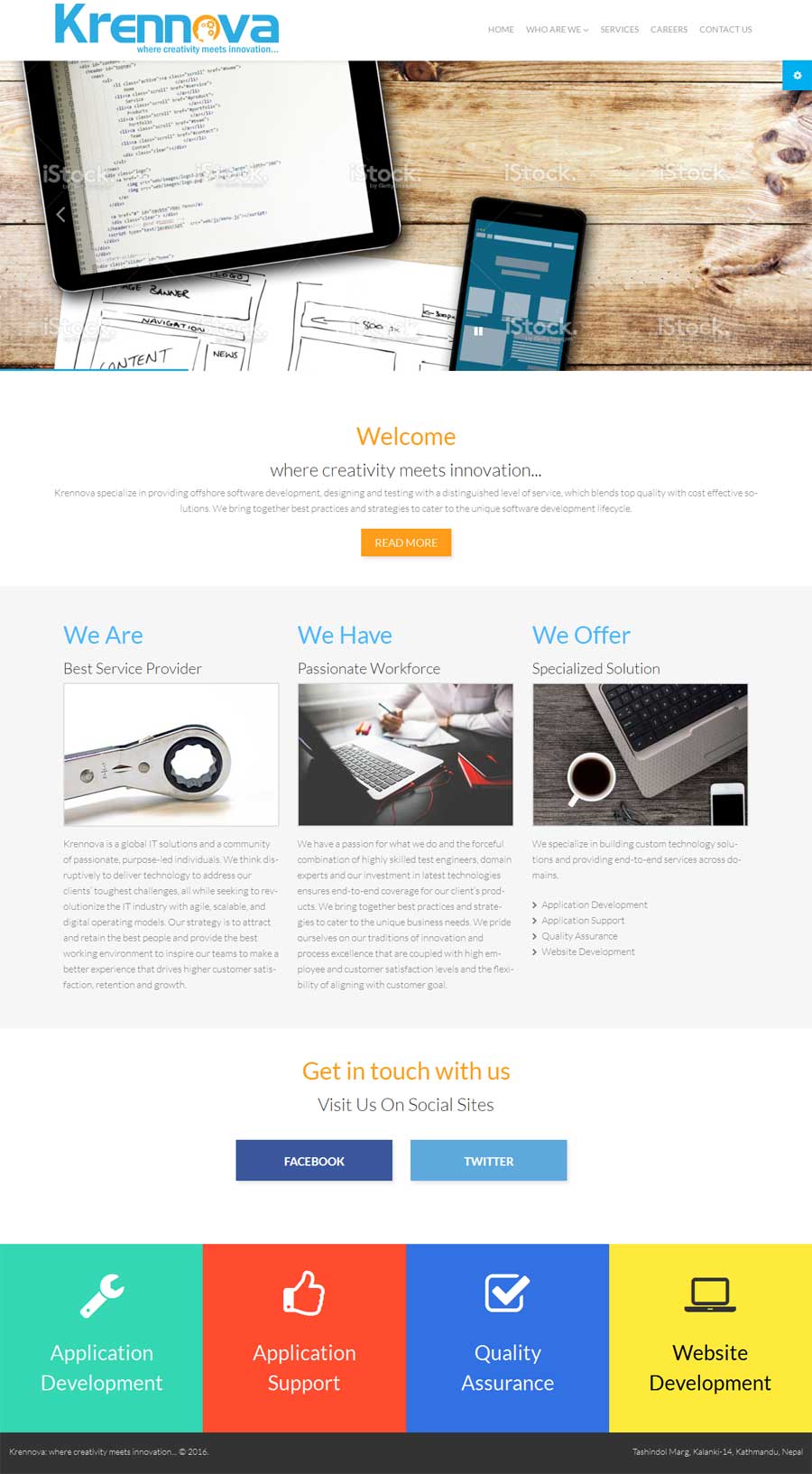This is a detailed screenshot, likely taken from a tablet, of the homepage of a website for a company named Crennova. The brand name "CRENNOVA" appears prominently at the top in blue, with the exception of a red ‘O’ that contains the side silhouette of a person’s head. 

To the right of the brand name, there are several navigation categories: "Home," "Who We Are," "Services," "Careers," and "Contact Us."

Beneath these categories is a large rectangular box displaying an image. The image showcases a wooden tabletop viewed from an angle, featuring a tablet resting on it. The screen of the tablet displays a page listing various items.

Adjacent to the tablet, there is an Android phone with a black border. The phone screen shows a blue background with some gray boxes. Partial visibility of a white paper positioned under both the tablet and phone reveals black writing and shapes. Key elements on the paper include the words "navigation," "banner," "content," and an orange text that reads "Welcome" beside the phrase "Where creativity meets innovation." There is also a segment discussing Crennova and an "Read more" button in an orange rectangular box.

Below this section is a gray rectangular box divided into three categories. 

1. **"We Are"**: Labeled as "Best Service Provider," illustrated with a picture of a wrench. The accompanying text describes Crennova as a global IT solutions provider and a community of passionate, purpose-driven individuals.

2. **"We Have"**: Defined as having a "Passionate Workforce," accompanied by an image of a laptop on a black table and a man in a dress shirt in the background.

3. **"We Offer"**: Highlighted as providing "Specialized Solutions." The image shows a top-down view of a laptop with a cup of black coffee, a cell phone with a white case, and a pair of glasses on a gray wooden table. The text speaks to Crennova's expertise in creating custom technology solutions and offering comprehensive services across various domains.

Under these sections, there is a prompt "Get in touch with us" followed by icons linking to Facebook and Twitter.

At the bottom of the page, there are four colorful square tabs with corresponding icons and categories:

1. A green square labeled "Application Development" with a wrench icon.
2. A red square marked "Application Support" with a thumbs-up icon.
3. A blue square titled "Quality Assurance" with a checkmark icon.
4. A yellow square named "Website Development" with a laptop icon.